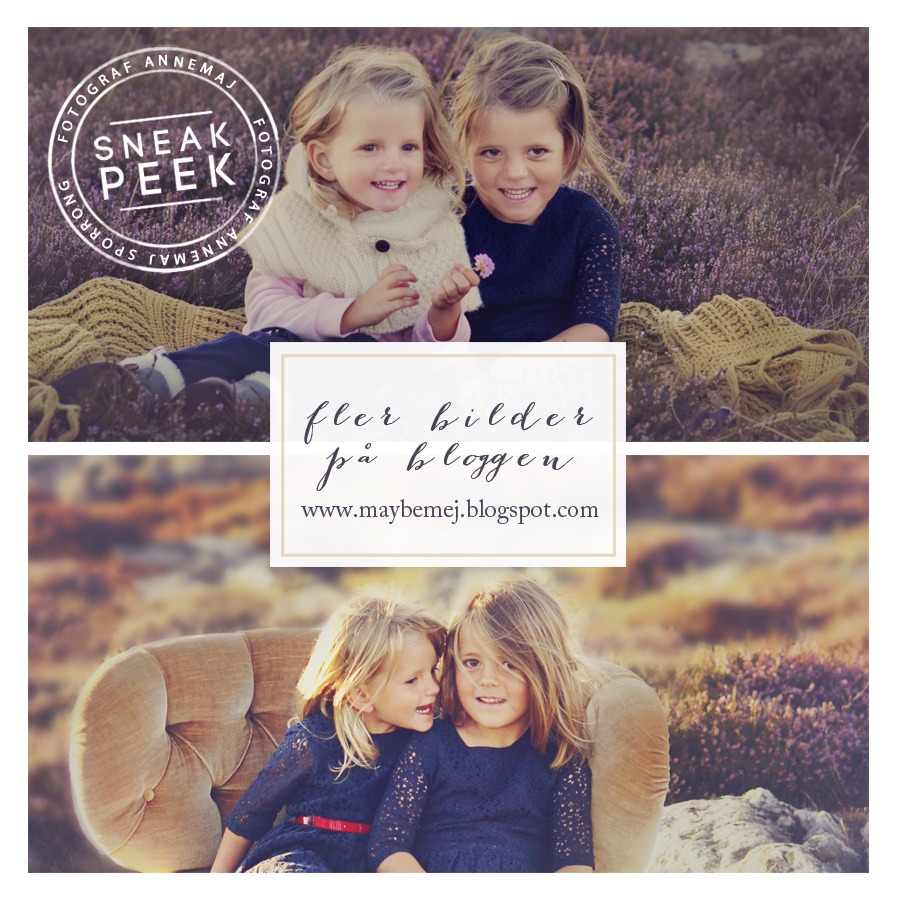This photograph consists of two side-by-side images featuring two young girls, most likely sisters, in what appears to be a professional photoshoot. The top image shows the girls, aged around three to five years, sitting on a moss green knitted blanket in a grassy field. They are wearing white cardigan sweaters and blue jeans, perhaps engaging with a flower or each other in a candid, natural pose. A circular logo in the upper left corner of this image contains the words "Photograph An-mah-juh-spor-on" and "sneak peek."

The bottom image showcases the same two girls sitting on a tan tufted chair, still in the same grassy field. This time, they are dressed in navy blue dresses, and their hair is styled differently. Between the two images, a white rectangular label centrally placed reads "Fleur Bilder Pabloggen" followed by the URL "www.maybemej.blogspot.com" in white lettering, which adds a cohesive professional touch to the overall composition. 

The entire setup, featuring yellowish-brownish cushions and the natural outdoor setting, evokes a warm, candid feel while maintaining a professionally polished look, highlighted by the branding and website information, as if previewing a set of high-quality family photographs.